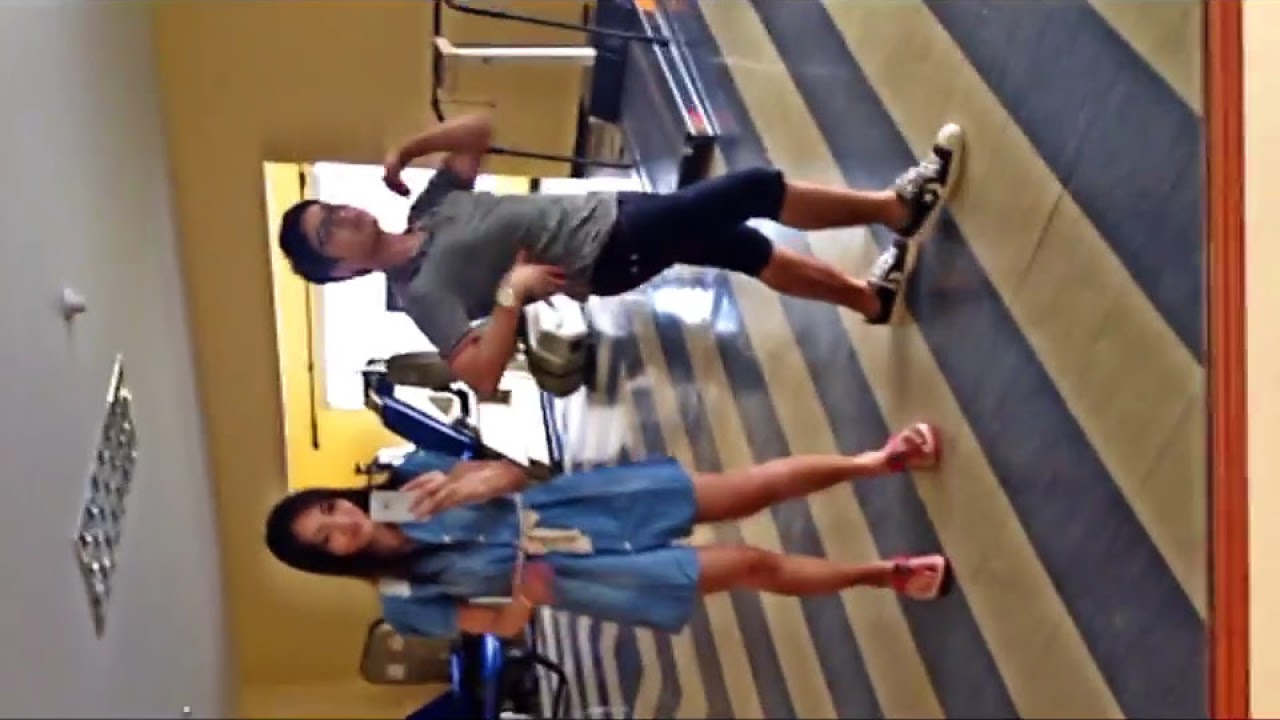The sideways image depicts a slightly blurry scene set in a gym with yellow walls, a white ceiling, and a blue and white striped mat covering the floor. Sunlight streams in through a window accented with a wooden border. In the image, two young adults stand on the mat. The boy, positioned on the right, sports a gray shirt, dark blue knee-length pants, a gold wristwatch, and black and white tennis shoes. He strikes a flexing pose with one hand raised, showing off his black hair and glasses. The girl on the left wears a blue short dress with a white ribbon around the waist, dark hair, and sandals. She focuses on a white cellphone in her hand. Gym equipment, possibly including a treadmill, is visible in the background. The ceiling also features a metal vent.